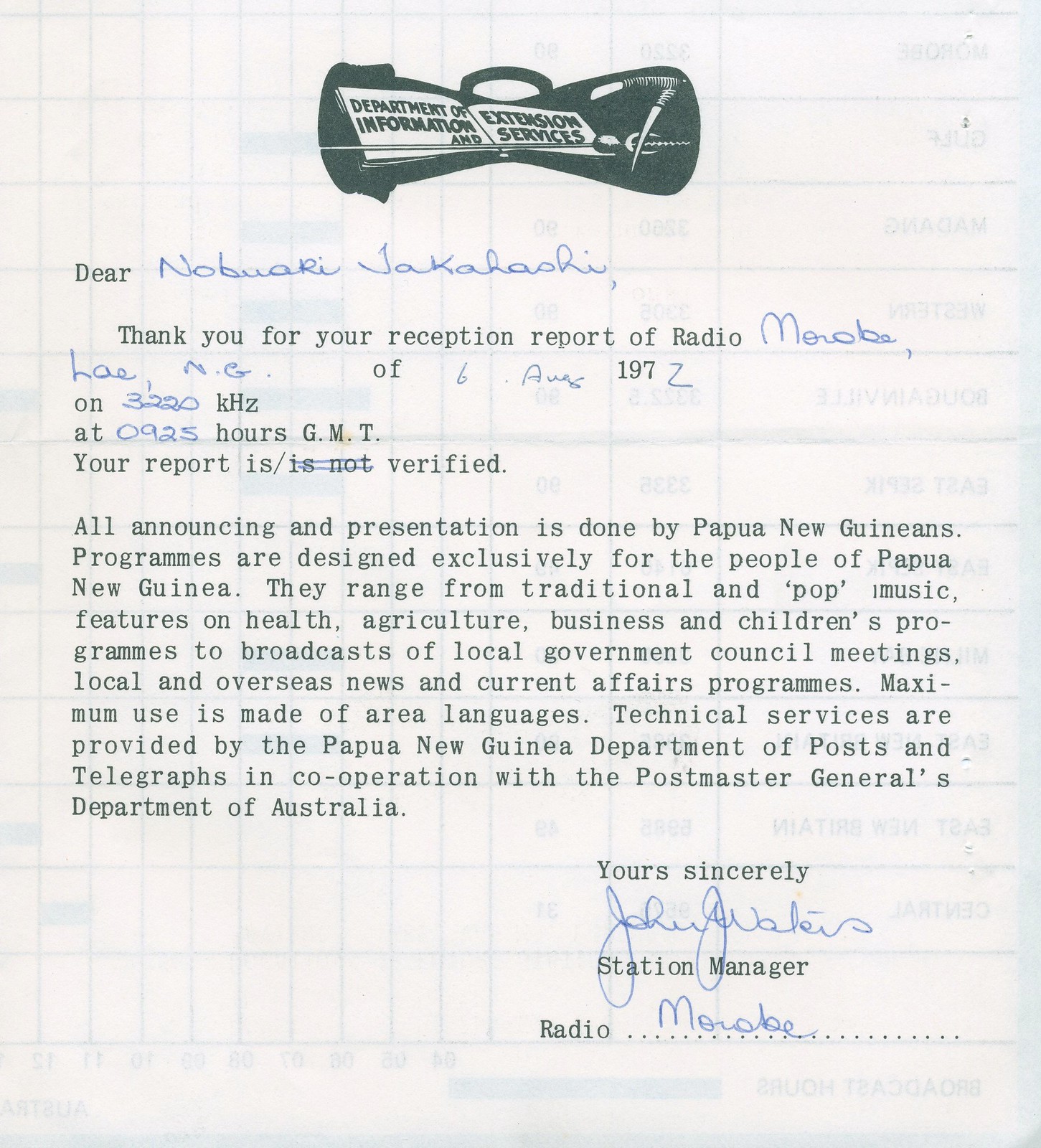This photograph showcases a typewritten letter from the Department of Information and Extension Services, prominently featuring their logo at the top. The logo consists of a white book inside a dark green bag-like design. The letter, addressed to Nobuaki Jakahashi, is dated 6th August 1972 and acknowledges a reception report of Radio Morobe on 3220 KHZ at 0925 hours GMT. The letter confirms the report's verification and elaborates that all announcing and presentation duties are performed by Papua New Guineans, with programs tailored exclusively for the local population. These programs span a diverse range including traditional and pop music, health, agriculture, business, children's programs, local government council meetings, and both local and international news and current affairs. The typewritten text appears in black ink, while the recipient's name and certain details are handwritten in blue ink. The signature at the bottom reads 'Yours Sincerely, Stationmaster, Radio Morobe.' The background hints at a faint grid-like pattern, possibly from the back side of the paper, adding a textured, see-through perspective to the overall image.